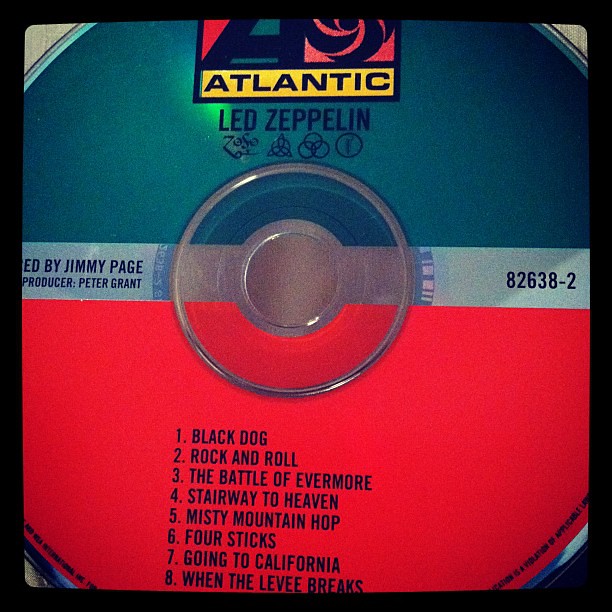The image is a close-up photo of an LP album, which prominently features a colorful disc at the center. The disc is divided into a green top half and a red bottom half, both sections containing black text. At the very top of the disc, in a yellow banner with black capital letters, it reads "Atlantic" along with their logo. Below this, it states "Led Zeppelin" accompanied by several symbolic logos, including Zoso, indicating it's Led Zeppelin's fourth album, also known as Led Zeppelin IV. In the middle of the record is a hole, and to the left of this hole, the text reads, “Produced by Jimmy Page; Peter Grant.” On the right side, the serial number "82638-2" is displayed. Below the hole, the track listing is clearly visible: 1. Black Dog, 2. Rock and Roll, 3. The Battle of Evermore, 4. Stairway to Heaven, 5. Misty Mountain Hop, 6. Four Sticks, 7. Going to California, and 8. When the Levee Breaks. The album is highly regarded as one of the best of all time, featuring distinctive artwork and typography.